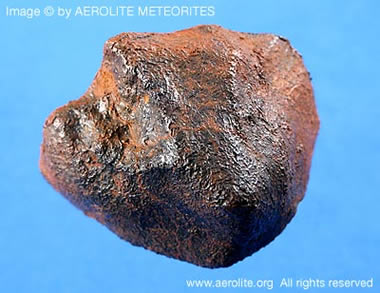The image features a striking meteorite set against a nuanced sky blue background that gradates from a light blue in the top left to a medium blue in the lower right corner. At the top left, there is a white caption that reads, "Image © by Aerolite Meteorites," accompanied by their symbol. The bottom right corner contains the text "www.aerolite.org. All rights reserved."

The focal point of the image is the meteorite itself, which is oblong and roughly textured, reminiscent of a space rock. Its surface is a beautiful amalgamation of colors; the top part exhibits a light rust-like orange, transitioning into a marbled texture blending with darker brown shades. Black hues appear in the lower portions, possibly accented with blue tinges. The rock has a slightly mitt-like shape, suggesting natural erosion or deliberate chipping, hinting at scientific examinations, such as testing for water erosion or life forms. This intricate marbling and rough texture make the meteorite both visually intriguing and scientifically significant.